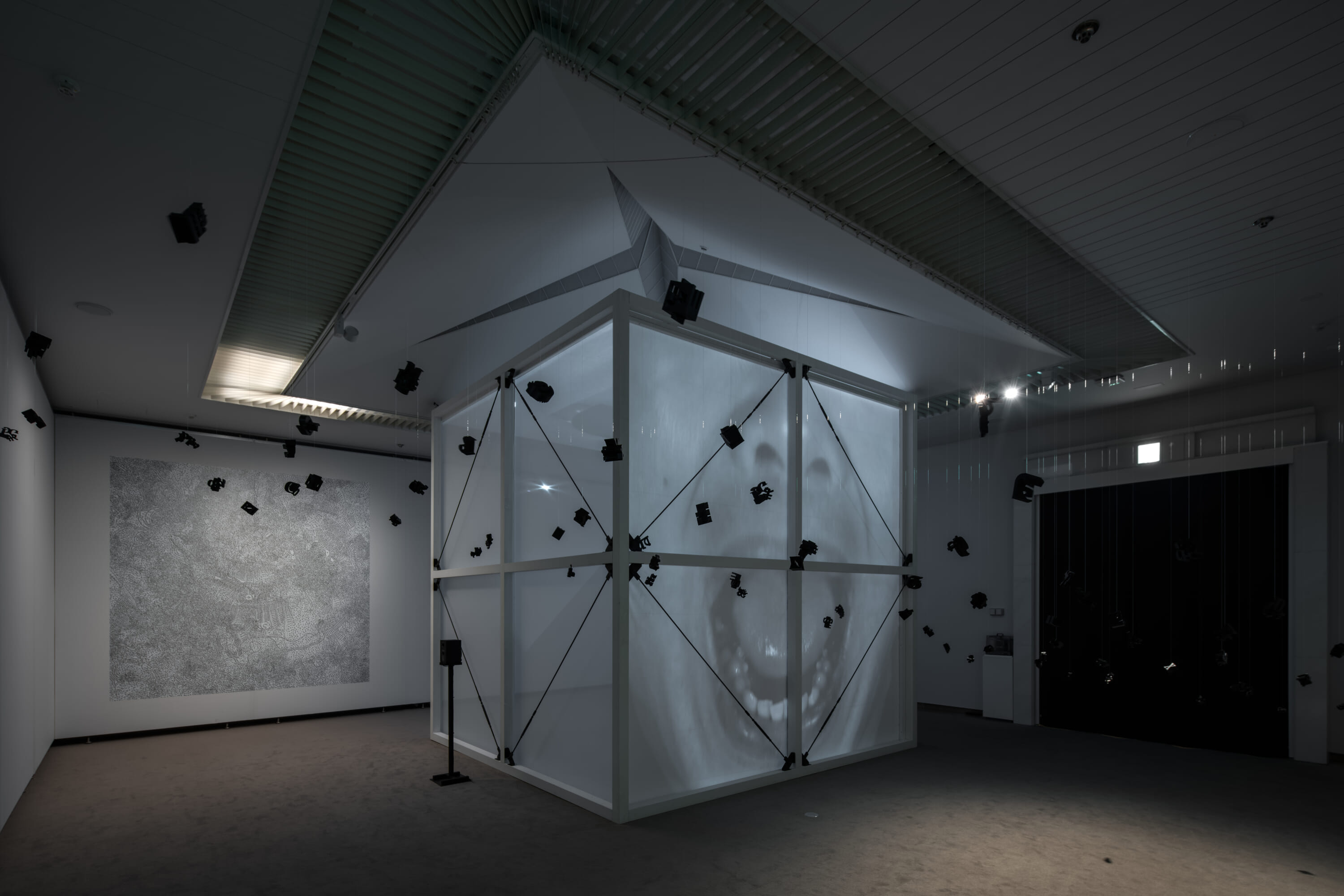The image depicts a computer-generated scene set within a modern art museum exhibit. The floor is composed of gray concrete, with a sleek, silver ceiling above. Dominating the center of the room is a large, transparent cubicle framed by white, diamond-patterned wiring. This central structure is adorned with a mesh-like, semi-transparent white fabric, giving it an ethereal quality.

On the right side of the cubicle, a striking black-and-white projection of a person's face is displayed, with the individual's mouth agape in a scream and nostrils flared, evoking a sense of fear and anguish. This grim visage adds a macabre element to the exhibit. The walls and ceiling of the space are scattered with enigmatic black devices or shapes, which could be cameras or simple geometric forms, enhancing the room's modern, avant-garde atmosphere.

To the right of the room, there is a large, dark portal-like doorway crowned with a glowing white exit sign, punctuating the stark, immersive environment. This meticulously crafted space, with its blend of transparent elements, dramatic projections, and minimalist design, epitomizes a cutting-edge art installation.